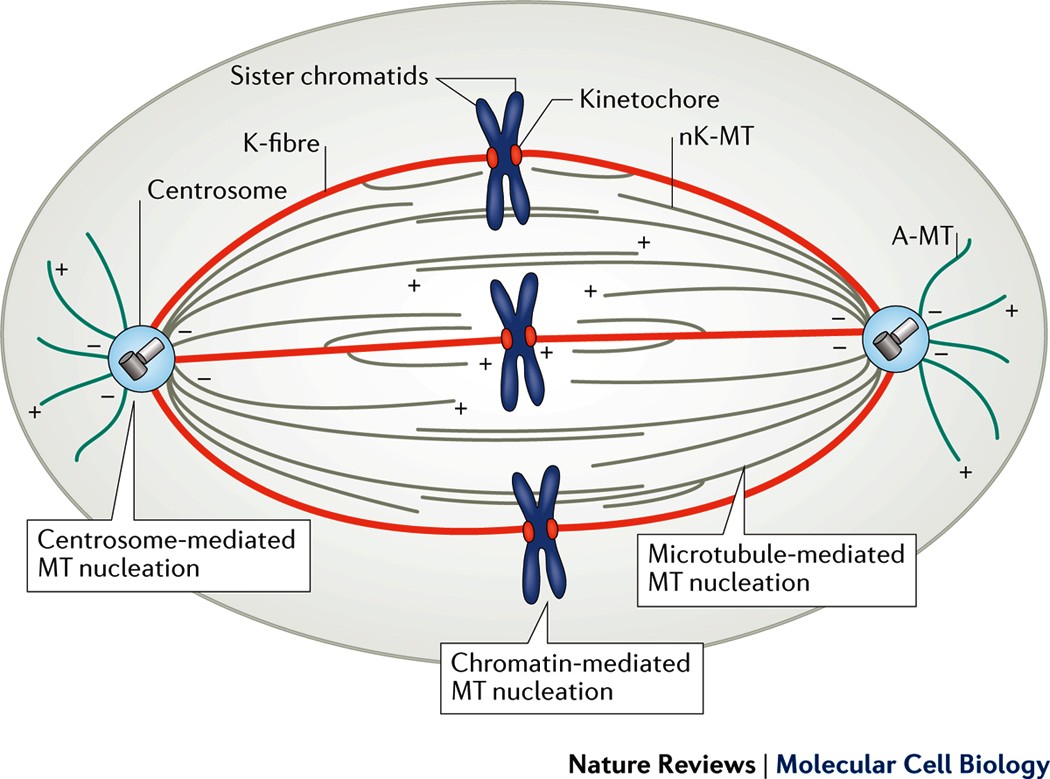The illustration is a detailed diagram related to molecular cell biology, prominently labelled "Nature Reviews Molecular Cell Biology" at the bottom. The main focus is an egg-shaped oval displayed in landscape mode, primarily in pale gray with a dark gray border. Inside the oval, the center features three large, dark blue X-shaped chromosomes. Each chromosome has red dots at the tips, marked as sister chromatids, and is connected by red lines indicating K-fibers.

At each narrow end of the oval, there are blue circular structures resembling hammers, representing centrosomes involved in centrosome-mediated MT nucleation, indicated by accompanying labels. The background of these circles is blue, with tan and silver tubes extending from them, likely depicting microtubules. Green wavy lines emanate from these tubes, providing additional detail to the depiction.

The diagram incorporates several other key elements, such as kinetochores (depicted in red adjacent to the X-shaped chromosomes) and labels for additional cellular components and processes, including NK-MT, microtubule-mediated MT nucleation, and chromatin-mediated MT nucleation. The harmonious use of colors—pale gray for the backdrop, dark and light blue, red, green, tan, and silver—enhances the clarity of this intricate diagram.